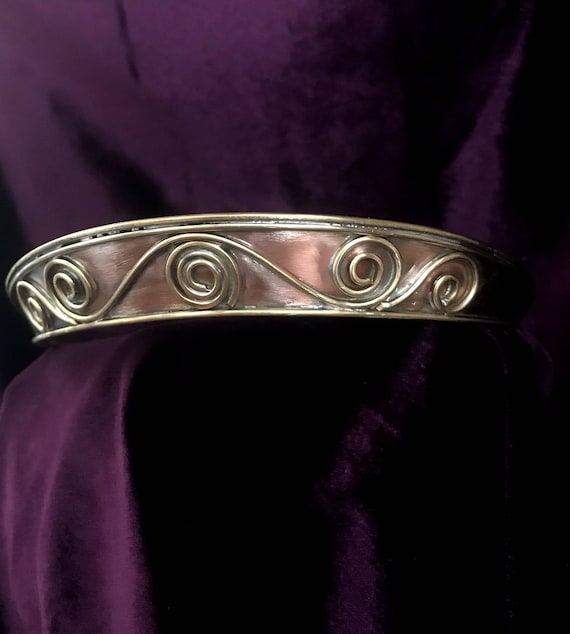The image showcases an elegant silver crown, potentially a tiara, adorned with intricate swirling designs that start as tight curls and gradually loosen as they extend. This metallic piece is set atop a purple velvet material, which appears to be tightly held in the middle by the crown, creating dark, heavy creases. The cloth exhibits a luxurious, deep purple hue, with noticeable shadows due to the lighting. The crown's detailed craftsmanship, with its shiny, classy appearance, suggests it might be an advertisement or auction listing. The overall composition, showing a side view of the crown, highlights its delicate and sophisticated design, akin to a headdress displayed on a velvet-lined holder.